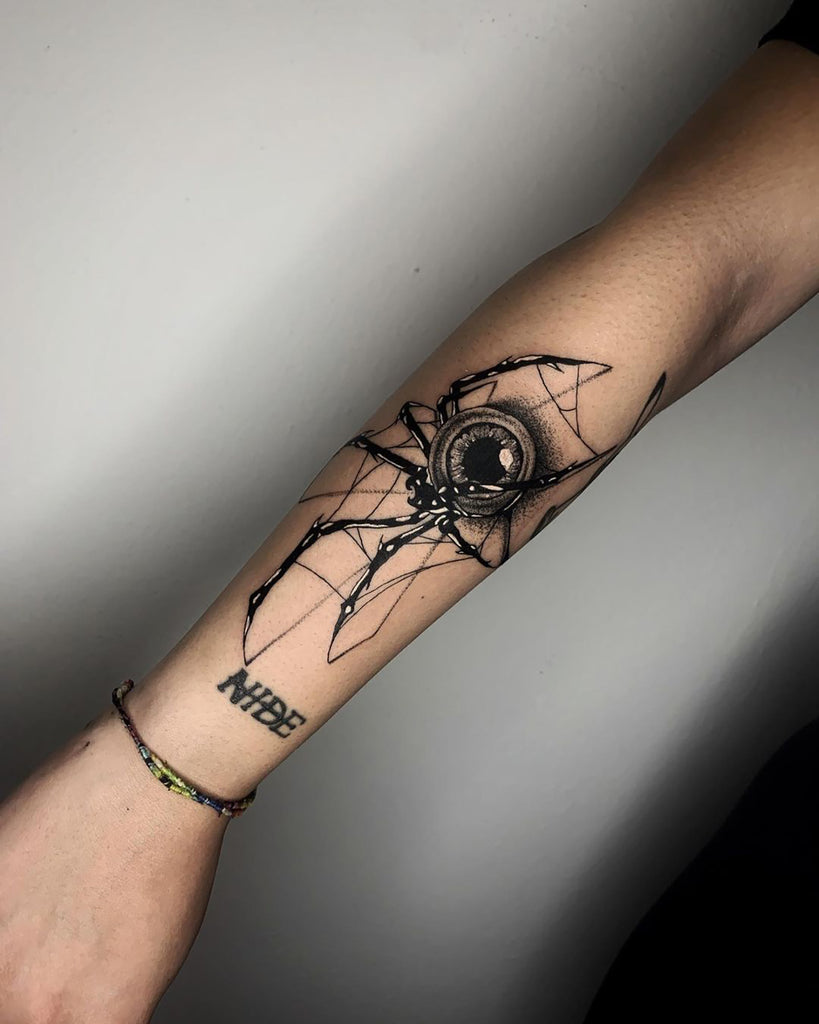This is a color photograph of a person's forearm adorned with a vivid black tattoo. The forearm extends diagonally from the upper right to the lower left, with the hand ending just before the fingers are visible. The background of the image is a gradient of gray to solid black at the lower right corner. The tattoo itself spans from just below the wrist to just below the elbow, depicting a thin, intricate spider with an eyeball as its body. The eye, detailed with an iris and pupil, is surrounded by black fuzz and web-like lines extending from the spider's legs. Above the spider, in the wrist area, is the text "N-I-D-E" with a line striking through it. The person wears a green and black, roped-style bracelet on their wrist.